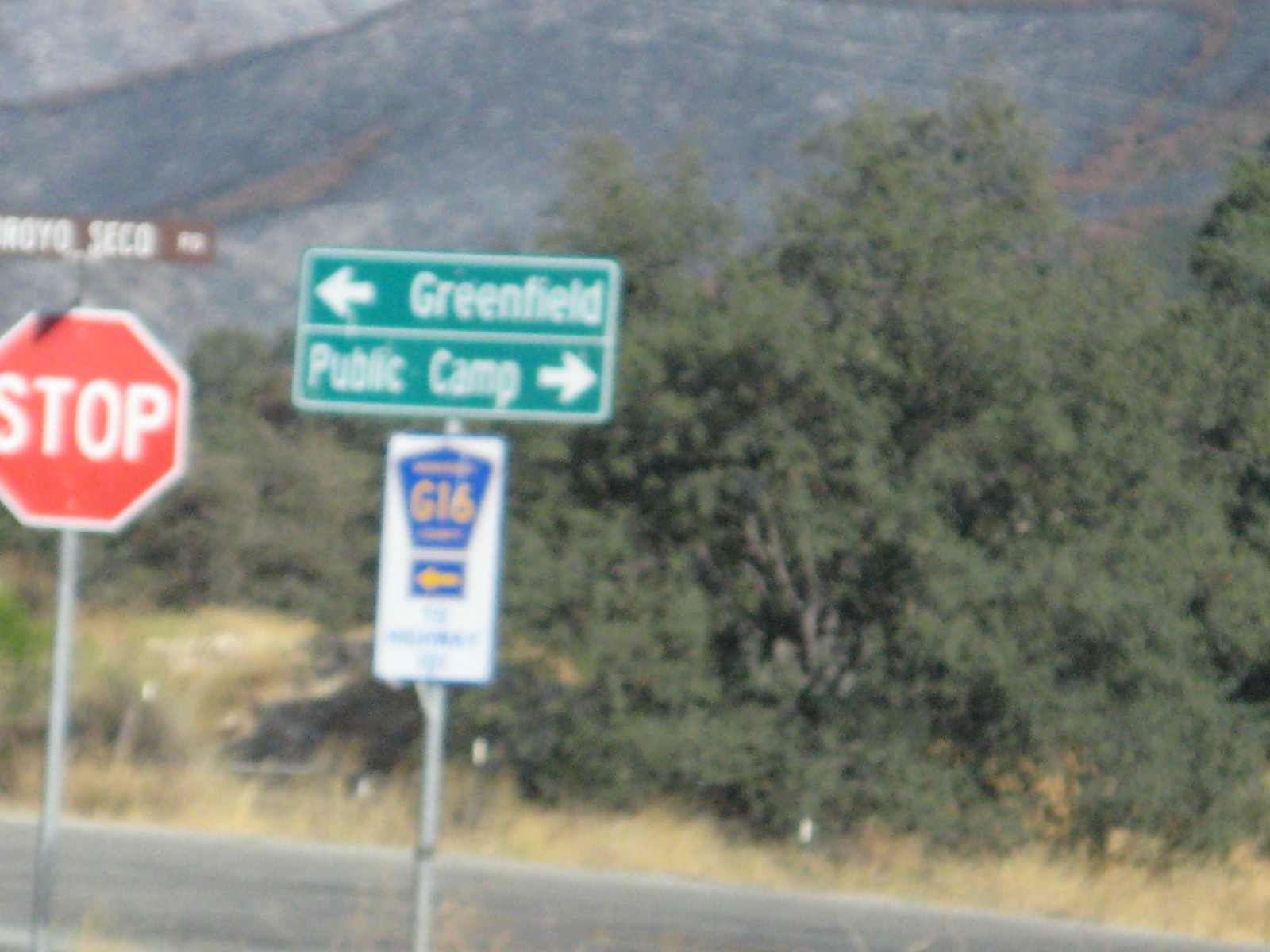This photograph captures a picturesque country road scene. On the left side, an octagonal red stop sign with bold white letters commands attention. Just above it, a rectangular brown sign with white lettering identifies a road, though the sign's text is partially blurred; the most legible part suggests the second word is "seed" followed by "road." Centrally located in the image, a green rectangular sign with white writing offers directions: "Greenfield" is marked at the top with a left-pointing white arrow, while "Public Camp" is indicated at the bottom with a right-pointing white arrow. Directly beneath this sign, a smaller white sign with a blue shield logo and gold writing reads "G16," accompanied by another gold arrow on a blue background pointing left. The image's lower portion showcases the road itself, framed by a few small trees that might be autumn olive trees, their leaves hinting at the season. In the background, a majestic landscape emerges, featuring a mountain or rock formation draped in hues of gray and rust, contributing to the serene and rustic ambiance of the scene.